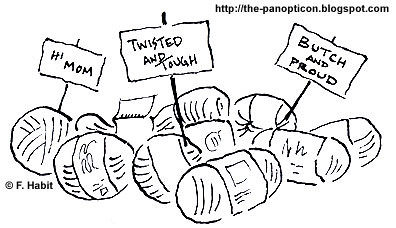This black and white illustration, reminiscent of a comic strip, features a group of yarn balls, each packaged with thin cardboard bands. There are six yarn balls in total, with four prominently in the foreground and two in the background. Each of the yarn balls holds a handwritten protest sign: the leftmost sign says "Hi Mom," the middle sign reads "Twisted and Tough," and the sign in the back right states "Butch and Proud." The caption "Copyright F. Habit" is typed on the left side of the image, while the URL "http://the-panopticon.blogspot.com" is written in the upper right corner.